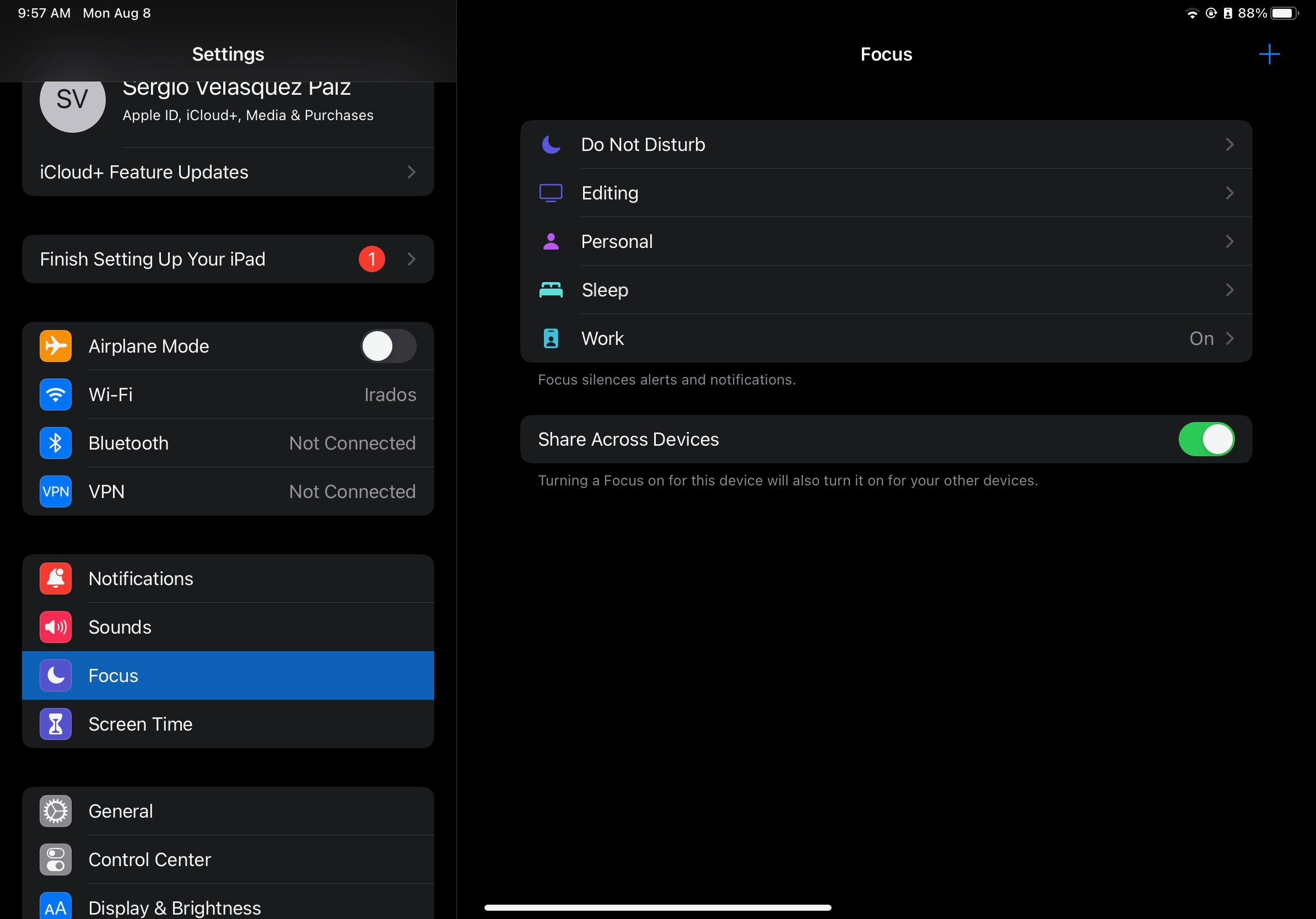The image is a detailed screenshot from the Settings app of an Apple device, likely an iPad, showcasing an elegant dark mode interface.

At the top left corner, the device's current time and date are displayed, indicating it is 9:57 AM on Monday, August 8th. On the top right corner, the screen indicates the device’s data and Wi-Fi strength, along with the battery life which is currently at 88%.

The left-hand side of the screen features a vertical column of selectable main options within the Settings app. At the top of this column is the username "Sergio Velasquez Pais," followed by various settings options like Wi-Fi, Bluetooth, and Notifications. These options are displayed in dark gray text, except for the 'Focus' setting, which is highlighted in blue, indicating it is currently selected.

The main focus of the screenshot is the detailed view of the 'Focus' settings, which occupy the right-hand side of the screen. At the top center, the word 'Focus' is prominently displayed in white text, followed by five additional options: Do Not Disturb, Editing, Personal, Sleep, and Work. These options are designed to customize the device's focus settings based on different activities or times of day.

Below these settings, there is another option labeled "Share Across Devices," allowing the user to synchronize the focus settings across all other Apple devices owned by Sergio Velasquez Pais. Overall, the dark mode theme and organized layout make the settings interface visually appealing and user-friendly.